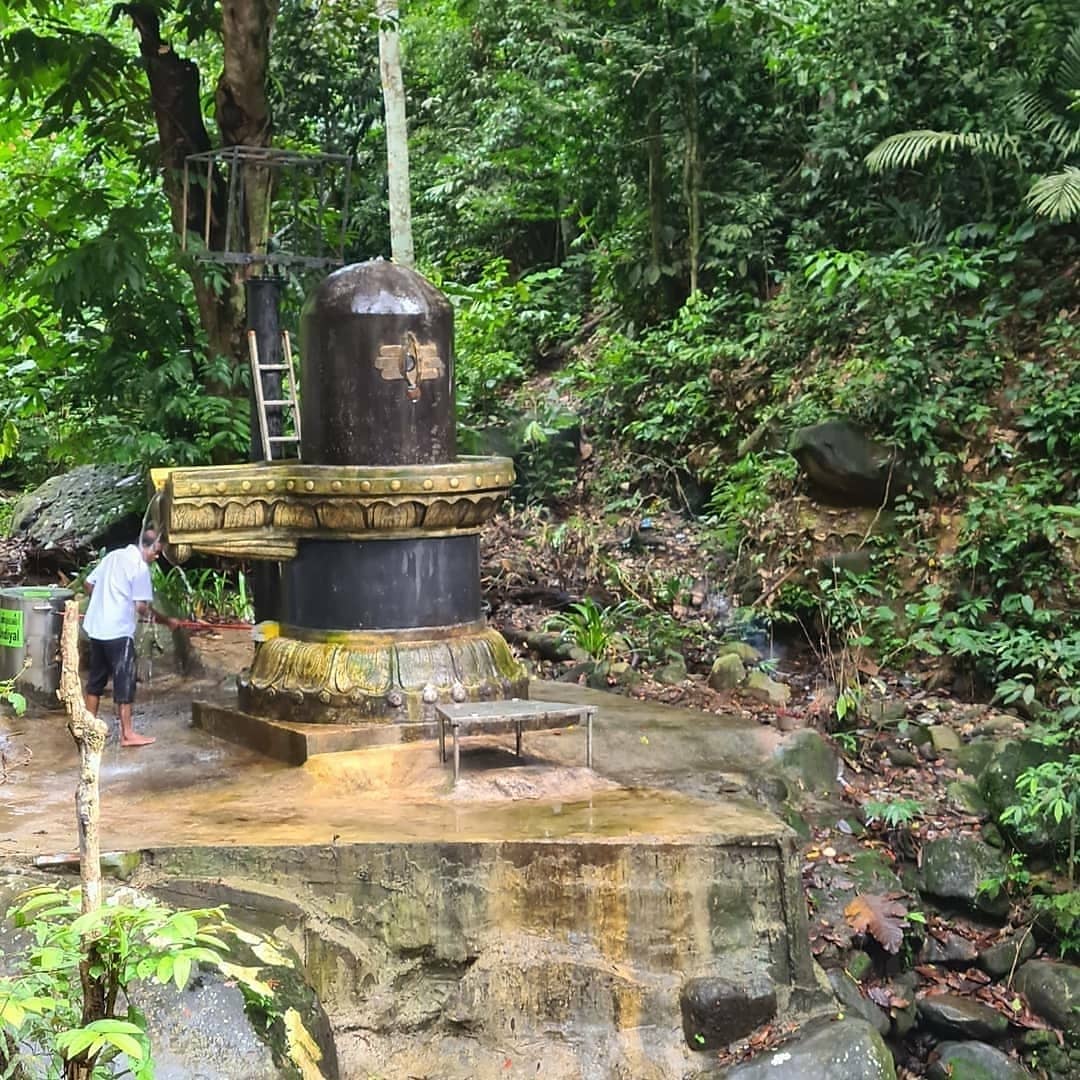In a lush, verdant rainforest, surrounded by an array of dark green and yellow foliage, stands an intriguing metal art installation. The upper half of the image is predominantly filled with dense green leafy trees and palm leaves. The top left corner features two tree trunks among the foliage, with a silver metal square holder in front of them and a black pipe descending into the forest floor. Leaning against this pole is a light brown wooden ladder. 

Centrally positioned is an unusual cylindrical structure, with a dome-like top and encased in a gold-like structure that gleams in the forest light. A dark brown tube, possibly rubber, runs vertically, adorned with a lighter birch-like trunk extending upwards to the center of the image.

At the base of this art piece, on a yellow cement platform, stands a barefoot man in a white short-sleeve shirt and black shorts. He holds a long red stick with a yellow mop at the end, seemingly cleaning or tuning the installation. The forest floor below him features dark wet rocks and scattered ferns, adding to the mystical, otherworldly ambiance of this unique scene.